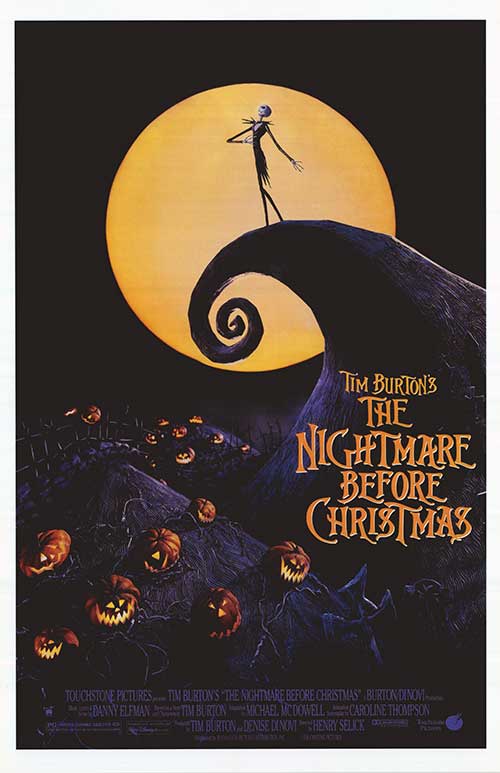This movie poster for Tim Burton's *The Nightmare Before Christmas* is dark and captivating, dominated by a large glowing orange moon set against a deep black night. The iconic character, Jack Skellington, dressed in his signature black suit, stands atop a twisted, swirled black hill that extends from the right side of the image. The landscape below is a haunting graveyard scene filled with glowing jack-o'-lanterns, illuminating the ground with an eerie light. A wooden fence runs through this spooky terrain, with one of the illuminated pumpkins hanging off it. The title, "Tim Burton's The Nightmare Before Christmas," is prominently displayed in a golden yellow font on the right side, while credits for notable contributors like Danny Elfman, Tim Burton, Michael McDowell, and Carolyn Thompson are listed at the bottom in purple text. The overall tonality of the poster is dark, emphasizing the nighttime setting and the film's haunting yet enchanting atmosphere.